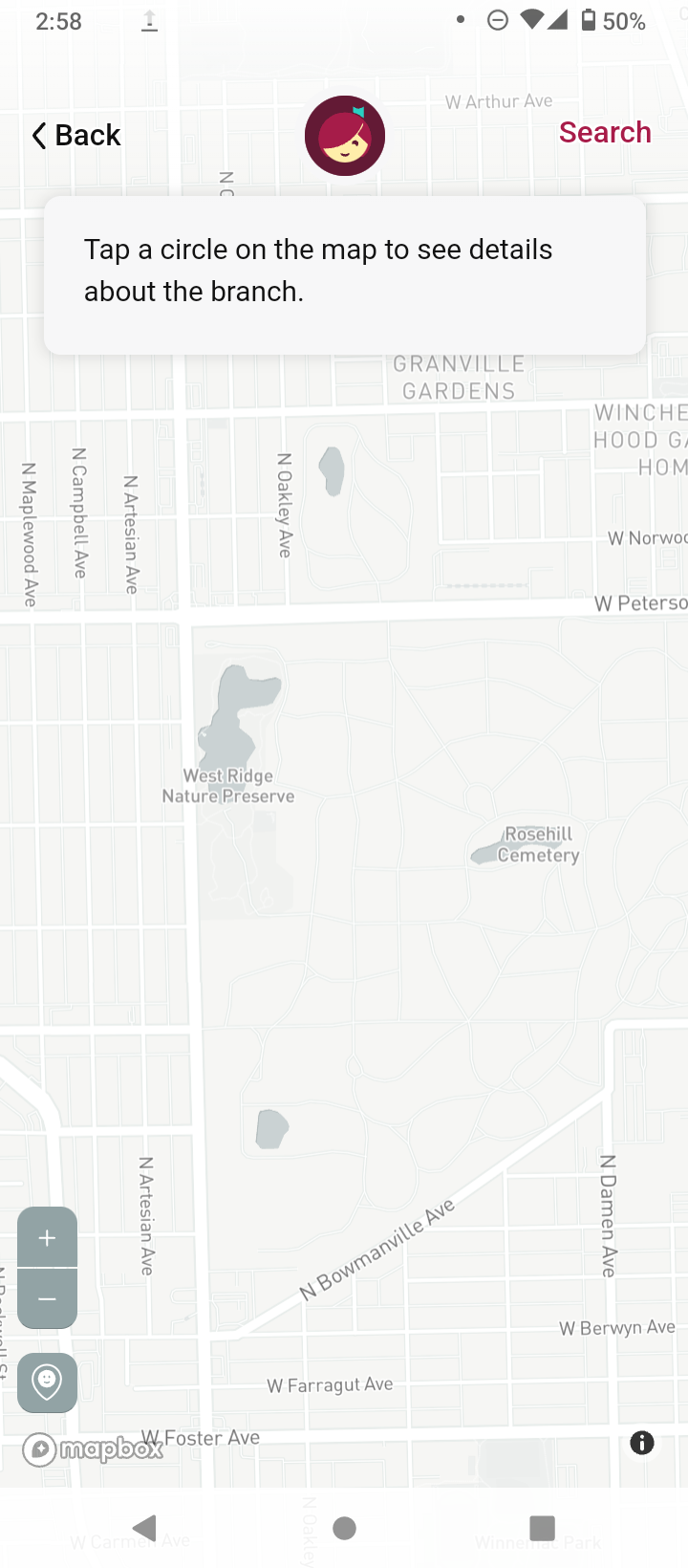The image displays a smartphone screen featuring a map from the Mapbox app, focused on an area with visible streets including West Foster Avenue, West Farragut Avenue, and North Bowmanville Avenue. Notable landmarks on the map include the West Ridge Nature Preserve and Rose Hill Cemetery. Additional streets shown on the map are North Oakley Avenue, North Artesian Avenue, North Campbell Avenue, and North Maplewood Avenue. A user icon, depicting a female avatar, is overlaid on the map, suggesting it is likely the phone belongs to a woman. The phone's status bar indicates the time is 2:58, the battery is at 50%, and the Wi-Fi is connected. An information icon is present in the lower right corner of the screen.